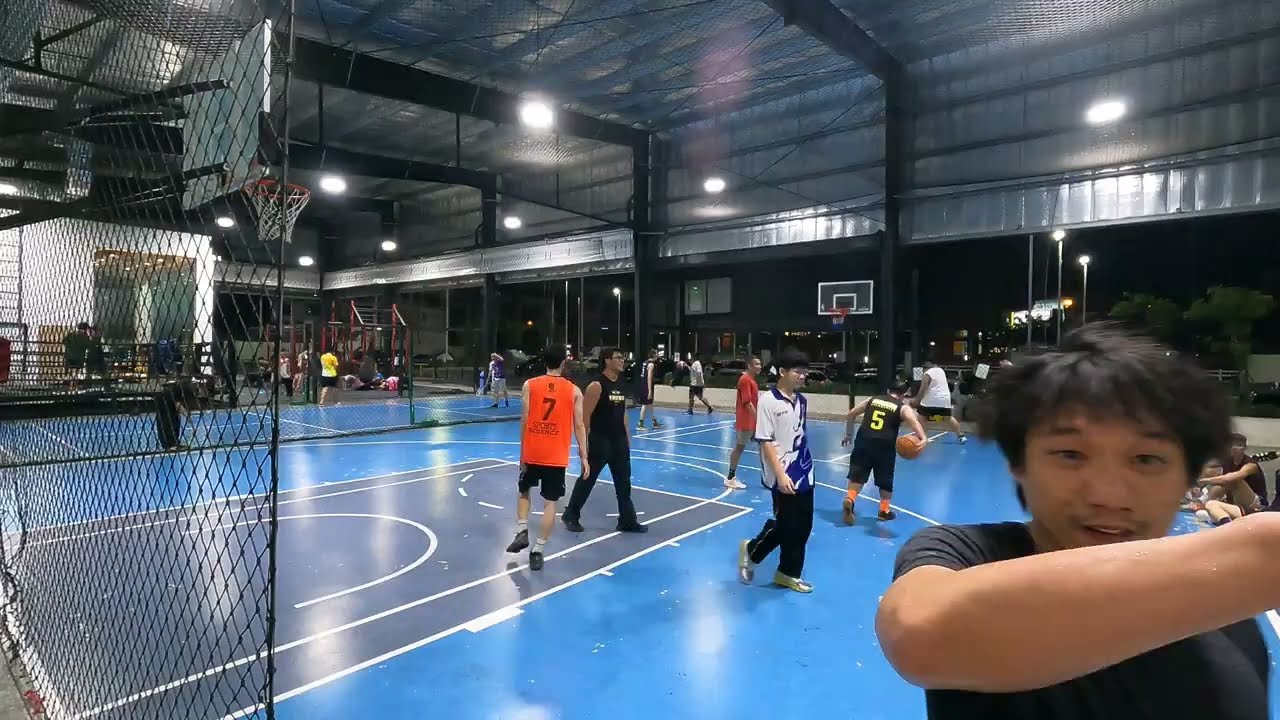The photograph captures a lively scene at a recreational center, featuring a basketball court as the central focus. The court itself is distinctively blue with turquoise accents marking the free throw areas. It's not a full-sized court but a smaller version, encompassed within a covered area with open walls, suggesting a half-indoor, half-outdoor setting. The nighttime backdrop reveals a dark sky, parking lot, and cars, enhancing the sense of an evening activity.

The spacious facility is bustling with activity. Around ten Asian individuals, all dressed in casual exercise attire rather than uniforms, are seen milling around the basketball court, engaging in recreational play. To the left, there's visible gym and workout equipment, alongside additional sports areas including another basketball court, a boxing ring, and a gymnastics zone.

Prominently close to the camera, in the bottom right corner, stands an Asian man in his 20s. He has black hair and is wearing a black t-shirt, partially smiling with one arm raised, almost obscuring his face. The ceiling above features metal sheeting with black beams, contributing to the rustic indoor-outdoor ambiance.